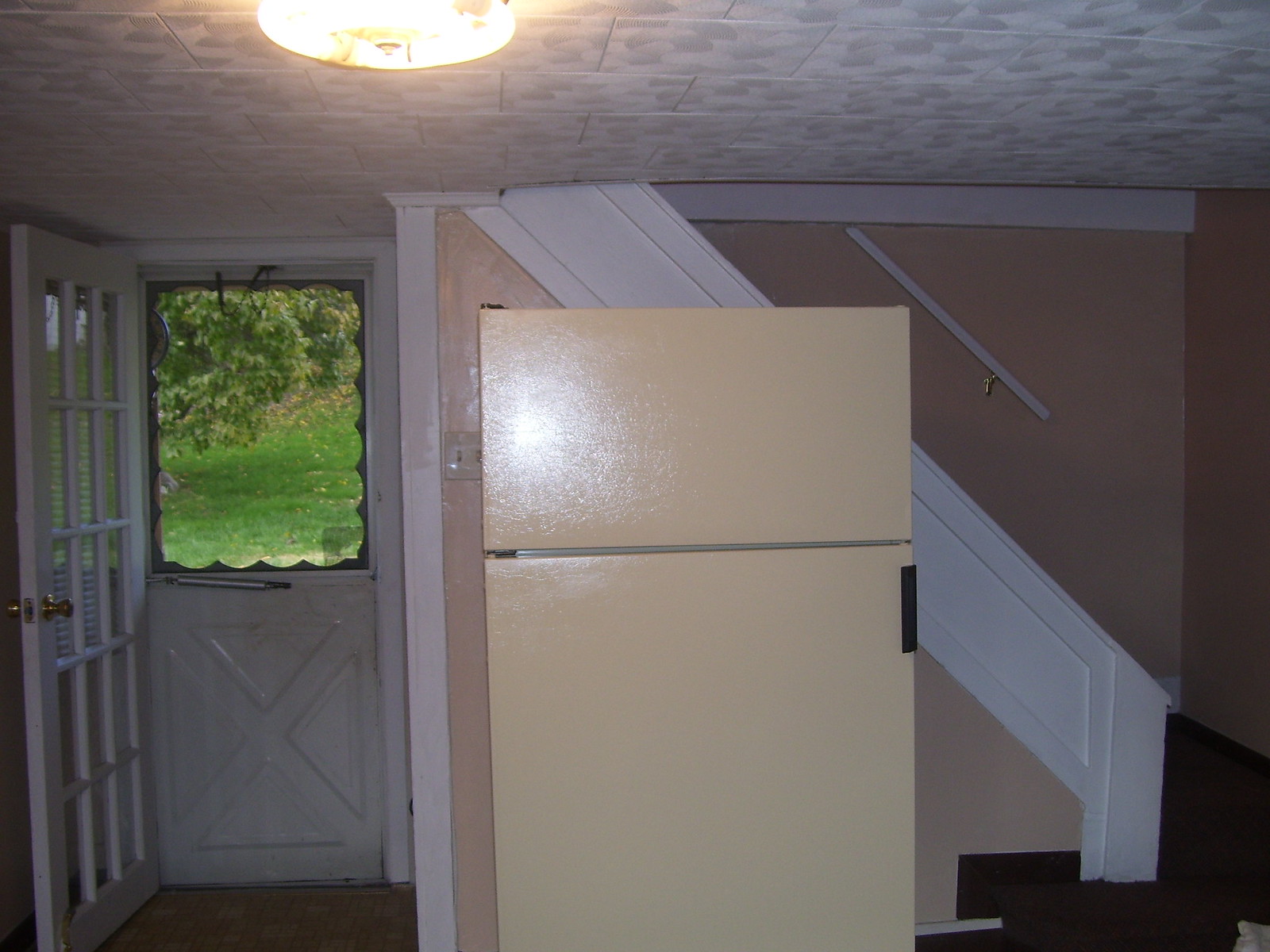This image depicts a cozy basement apartment with a low, white tiled ceiling featuring a seashell design. The focal point in the center, slightly to the left, is an older model refrigerator with a cream or tan finish. The top third of this clean unit is a freezer, complete with a small black handle on the right side for the fridge compartment. Behind the refrigerator, the wall is painted a soft peach color and features white trim. There’s also a white railing attached to the wall that leads up a staircase on the left, hinting at the upstairs area. To the far left, an open white wooden door with multiple "Brady Bunch-style" windows opens to reveal a white metal screen door. Through the doors, you get a glimpse of a green garden with branches, leaves, and grass visible but no tree trunk. The flooring between the areas is distinguished by a dark brown hue near the steps and a lighter wooden floor in front of the door.